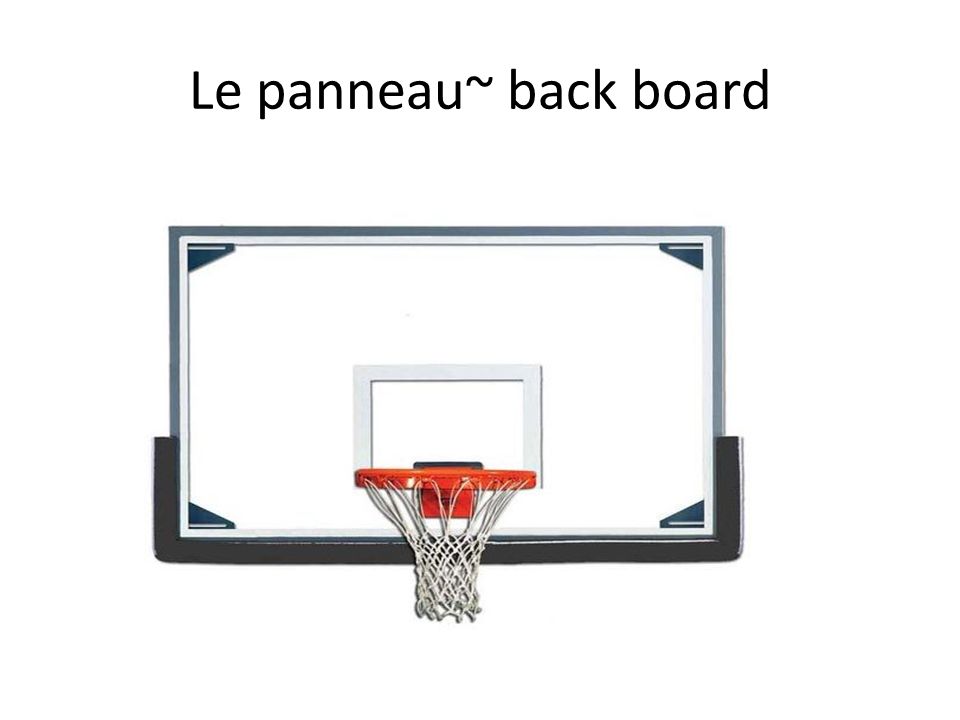The image is a digitally generated illustration of a basketball backboard and hoop, set against a white background with black borders that are thicker at the bottom. The backboard is depicted as clear glass with a white square centered above the hoop, which is an orange rim with a white net. The image includes gray or light blue lines outlining the backboard, with dark blue or gray reinforcing triangles in each corner. Along the bottom of the backboard runs a thicker black strip that extends slightly up the sides. The top of the image features the black-lettered text "Le Panneau Backboard," suggesting it may be part of an advertisement for this type of basketball backboard.